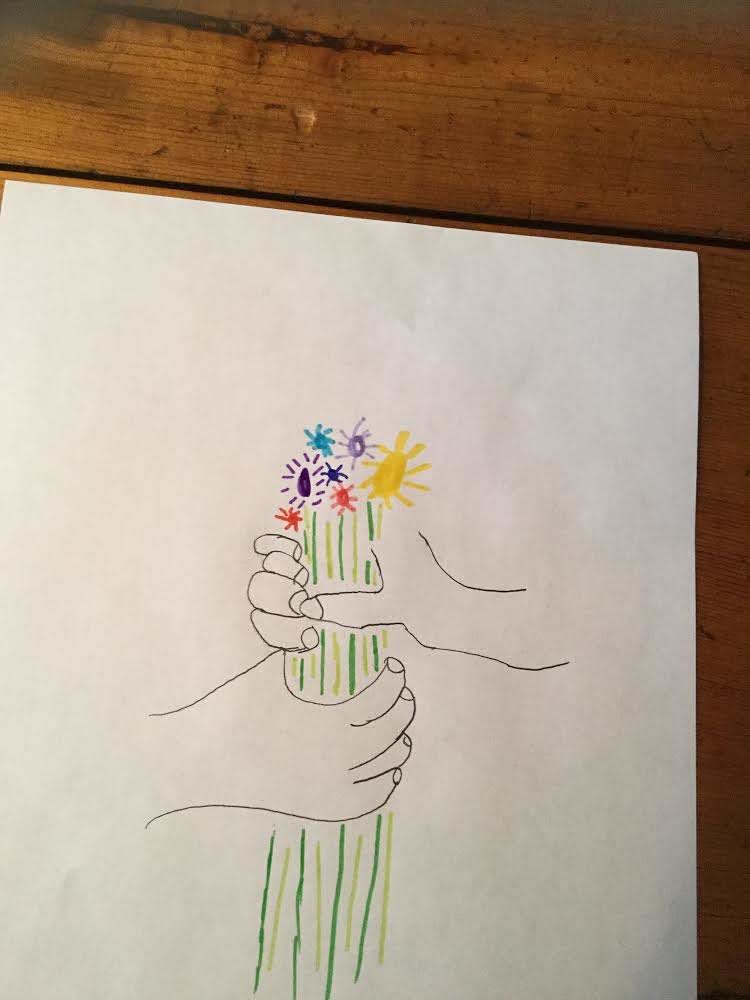A detailed close-up illustration showcasing two hands, seemingly belonging to different individuals, holding a vibrant bunch of flowers. The hand emerging from the left side of the scene grasps the lower portion of the flower stems, its front part tightly encircling the greenery. Meanwhile, a second hand, entering from the right, secures the upper section of the stems, with its fingers and thumb visibly wrapping around the top of the bouquet. The stems, numerous and vividly green, provide a striking contrast to the artistically rendered flowers above. The blooms, drawn with colorful markers, feature simple dot centers and whimsical marker lines as petals. This contrasts beautifully against the delicately penciled hands, which showcase fine details and expert shading.